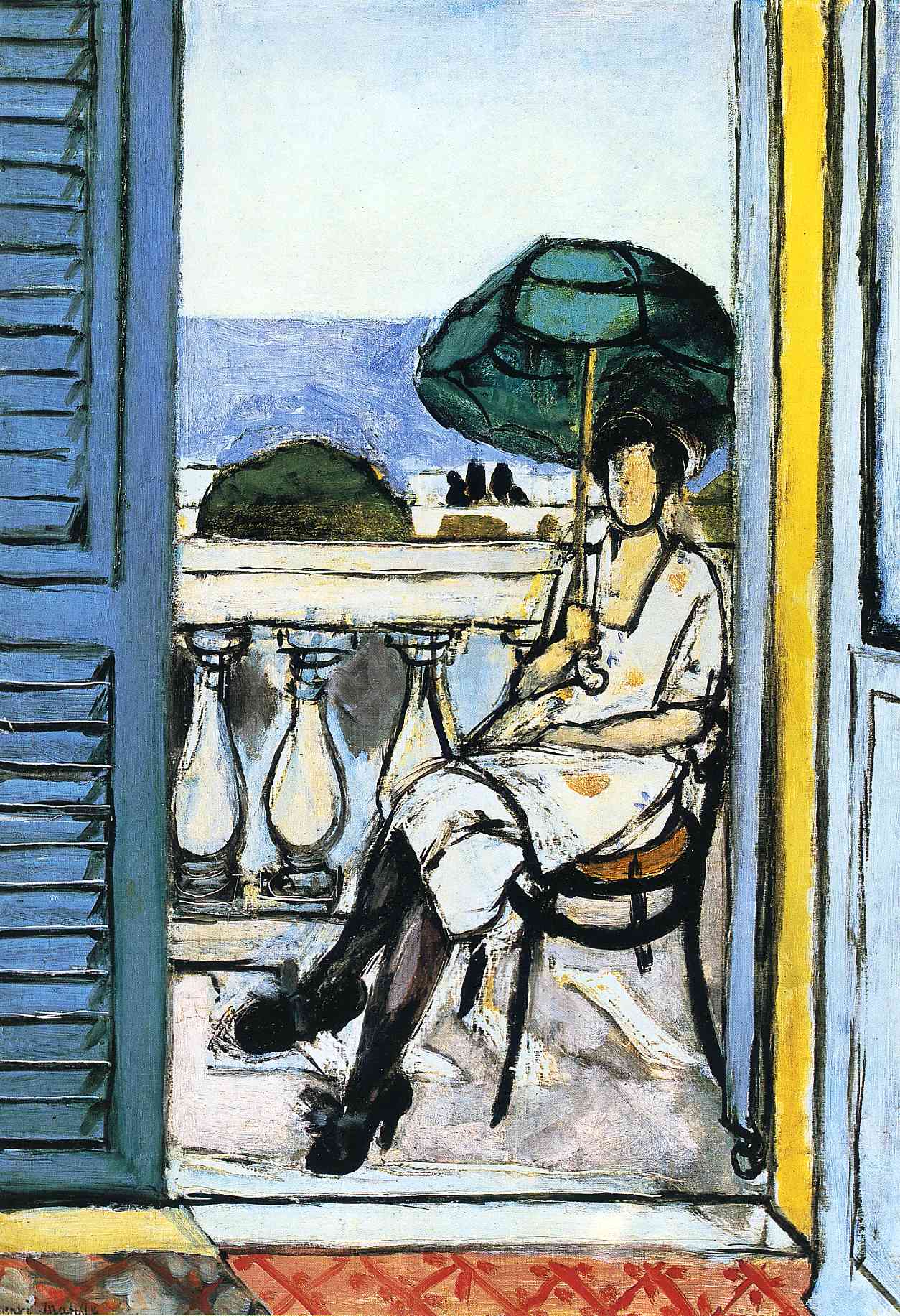In this vividly colored abstract painting, a woman is depicted sitting on a small circular stool on her porch or balcony. She's framed by a doorway, with a red patterned rug inside and blue shutters to the left. The woman is dressed in a white dress adorned with yellow flowers and outlined in thick black lines, paired with black stockings and black heeled shoes. She holds a green parasol with a gold handle in her right hand, shading herself as she sits. Her dark hair is pulled back, and she lacks facial features. The balcony is surrounded by white, obelisk-style balusters. Beyond the railing, a bright sky with light and deep blues and the green tops of distant trees can be seen, suggesting a tranquil, outdoor setting. The door frame is painted yellow and the door itself is blue, adding to the vibrant and dynamic color palette of the scene.